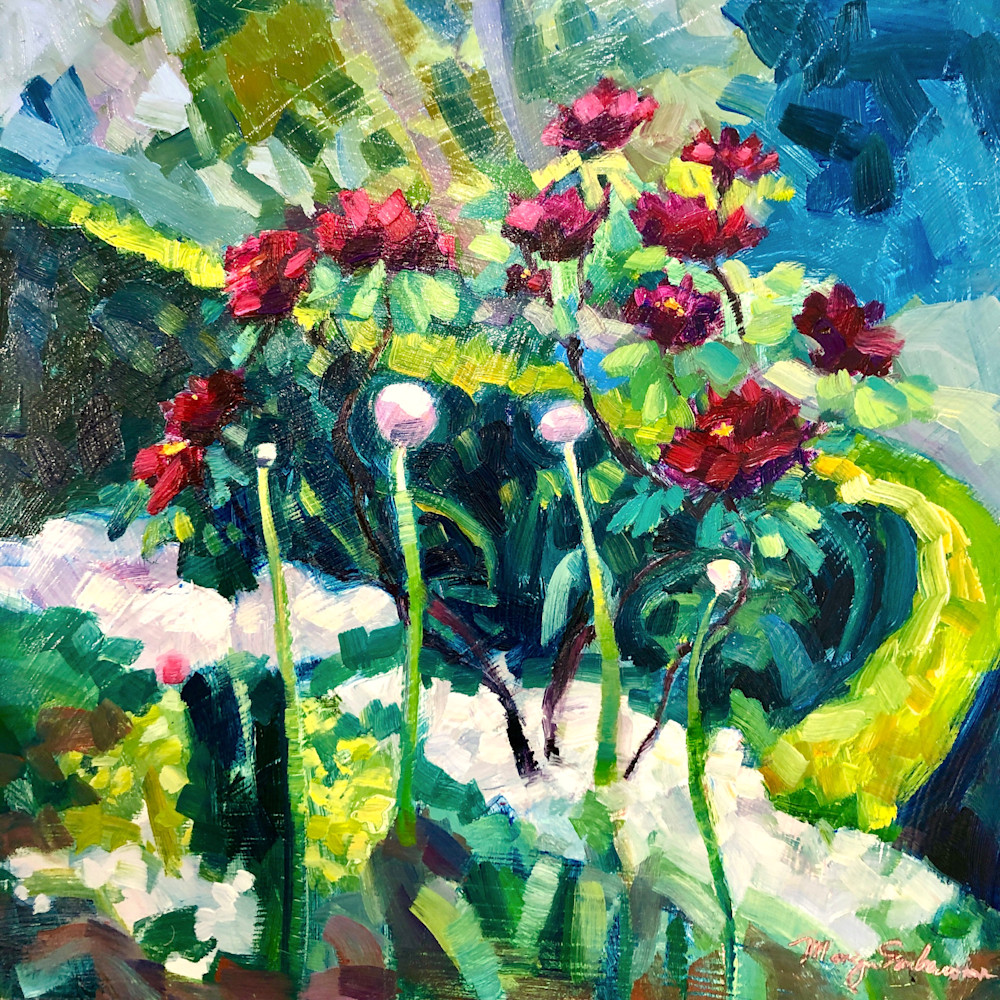This vibrant and abstract square painting features an intricate depiction of a rose bush bathed in a kaleidoscope of colors. The artist's cursive signature in red and white graces the bottom right-hand corner of the image. The upper portion of the artwork reveals a sky-like expanse with a significant blue patch on the top right, transitioning into an array of greens, yellows, and purples towards the center. The top left includes a combination of browns, greens, blues, pinks, and whites. A dynamic streak of lime yellow-green extends from the upper left, flowing diagonally downward to the middle right before curving back. Toward the center, the scene bursts with flora, showcasing large red flowers with yellow centers, accompanied by round pink buds on tall stems. Amidst this floral array, scattered yellow flowers and lush green foliage further enrich the scene. The lower portion features a row of whitish-pink extending from the middle left to the bottom right. Though abstract in nature, the painting vividly conveys the essence of its floral subjects under a sunny sky, creating a breathtaking and immersive visual experience.